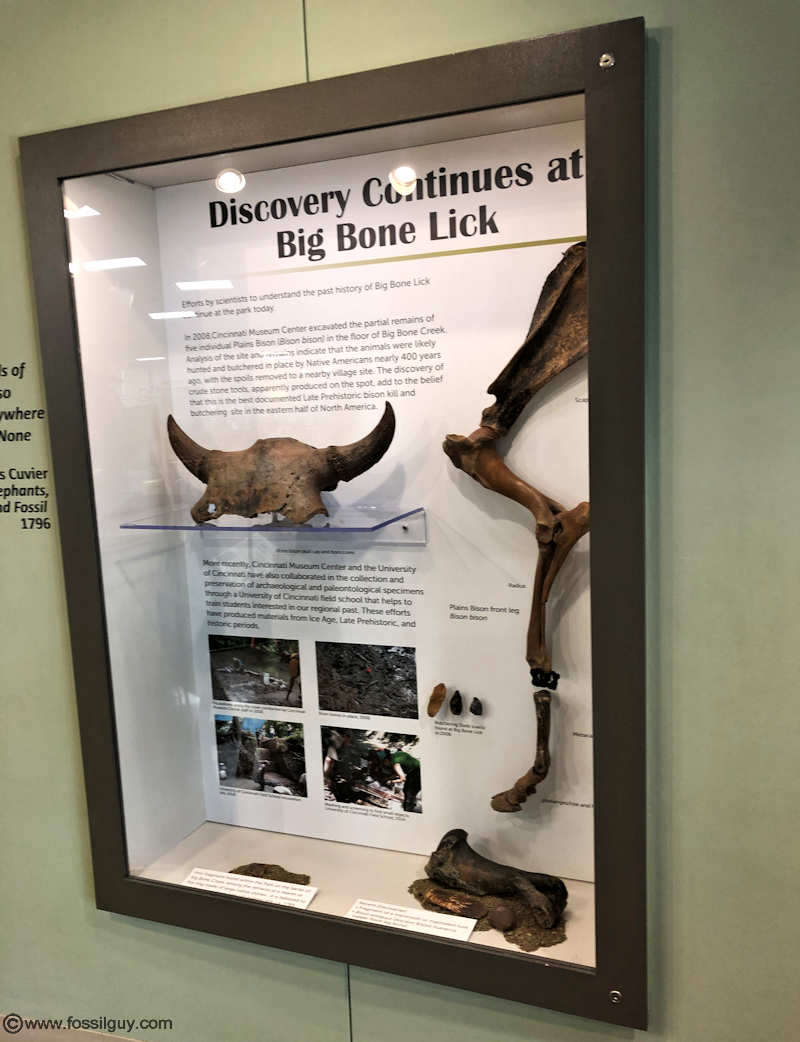This photograph features a detailed museum exhibit, prominently titled "Discovery Continues at Big Bone Lick," encased in a black-framed glass display. The background of the display is green, and reflections from ceiling lights are visible on the glass. Central to the exhibit is a descriptive document detailing ongoing scientific efforts to uncover past histories at Big Bone Lick. The document mentions the Cincinnati Museum Center's analysis of a bison skull fragment excavated from Big Bone Creek, though some of the text is difficult to read.

Within the display, various bone fragments are arranged, including a significant portion of an animal skull with two horns, potentially of a bison or an ancient bull. Accompanying the skull are three smaller bone fragments and two others at the very bottom, all labeled but unreadable from the image. Below the primary artifacts, four images depict the excavation process. On the left side of the frame, partially readable background text includes words like "where," "none," "Cuvier," "fossil," and "1796," likely referencing scientists and historical details associated with the exhibit. The lower left corner of the display includes the watermark "www.fossilguy.com," suggesting the source or contributor of the exhibit.